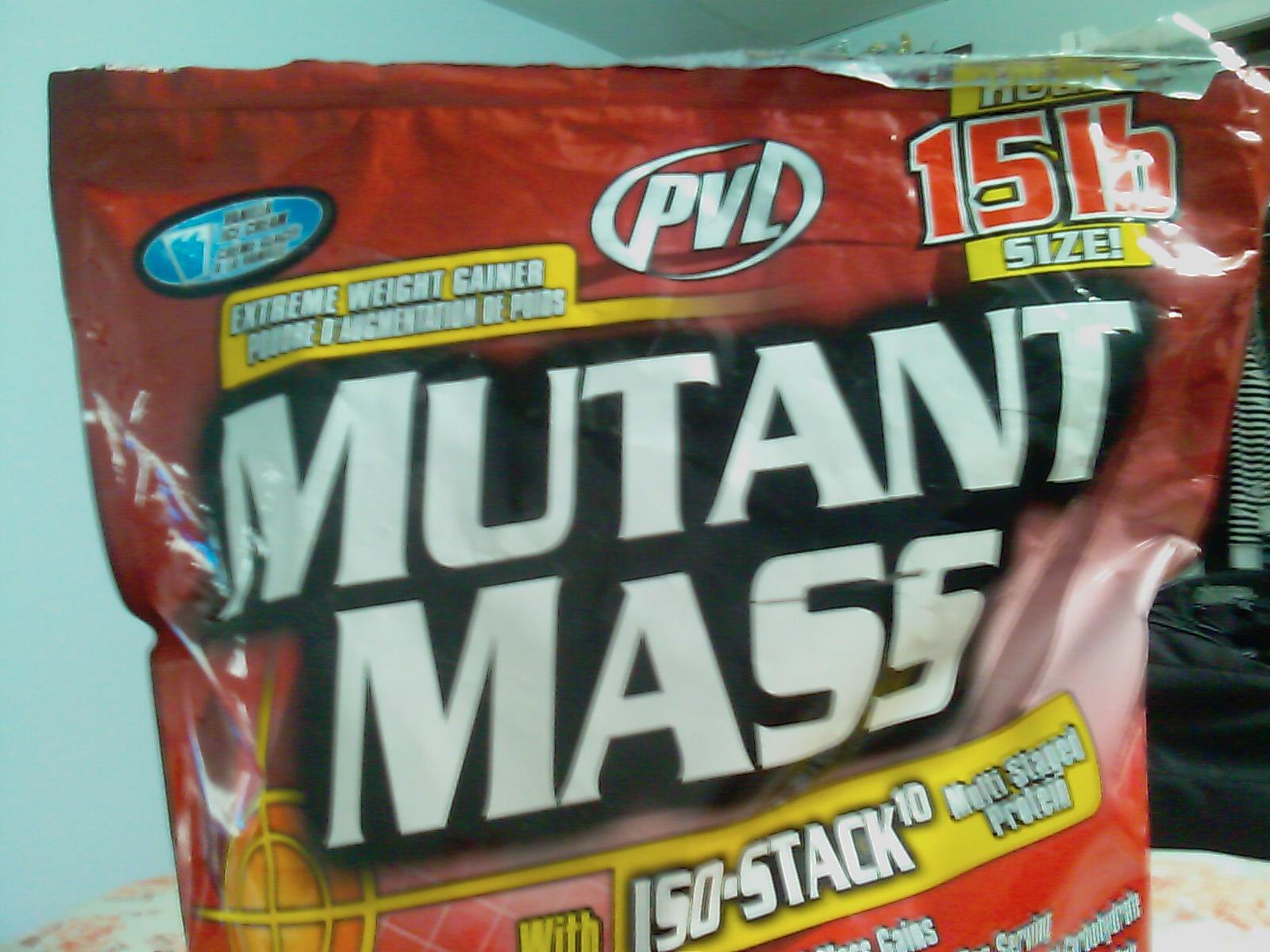The image captures a close-up view of a large rectangular package situated indoors, likely within the confines of a home. The setting appears to include furniture or bedding with a rich floral design in the background, though the exact room remains indistinct—potentially a bedroom. The walls, possibly reflecting soft blue hues due to ambient lighting, and the suggestion of window blinds towards the right-hand side add to the cozy, domestic atmosphere. 

Dominating the scene is a prominently displayed red package of "Mutant Mass." The branding "PVL" is visible, and emphasizes a sizeable 15-pound container of an "extreme weight gainer." The striking title "Mutant Mass" is presented in large, bold white letters set against partial black backgrounds. Below, the package is adorned with various informational texts, segmented into strips of yellow and red with white lettering detailing product specifics. An additional, indistinct black object rests in front of the floral pattern in the backdrop, contrasting the otherwise brightly colored scene.